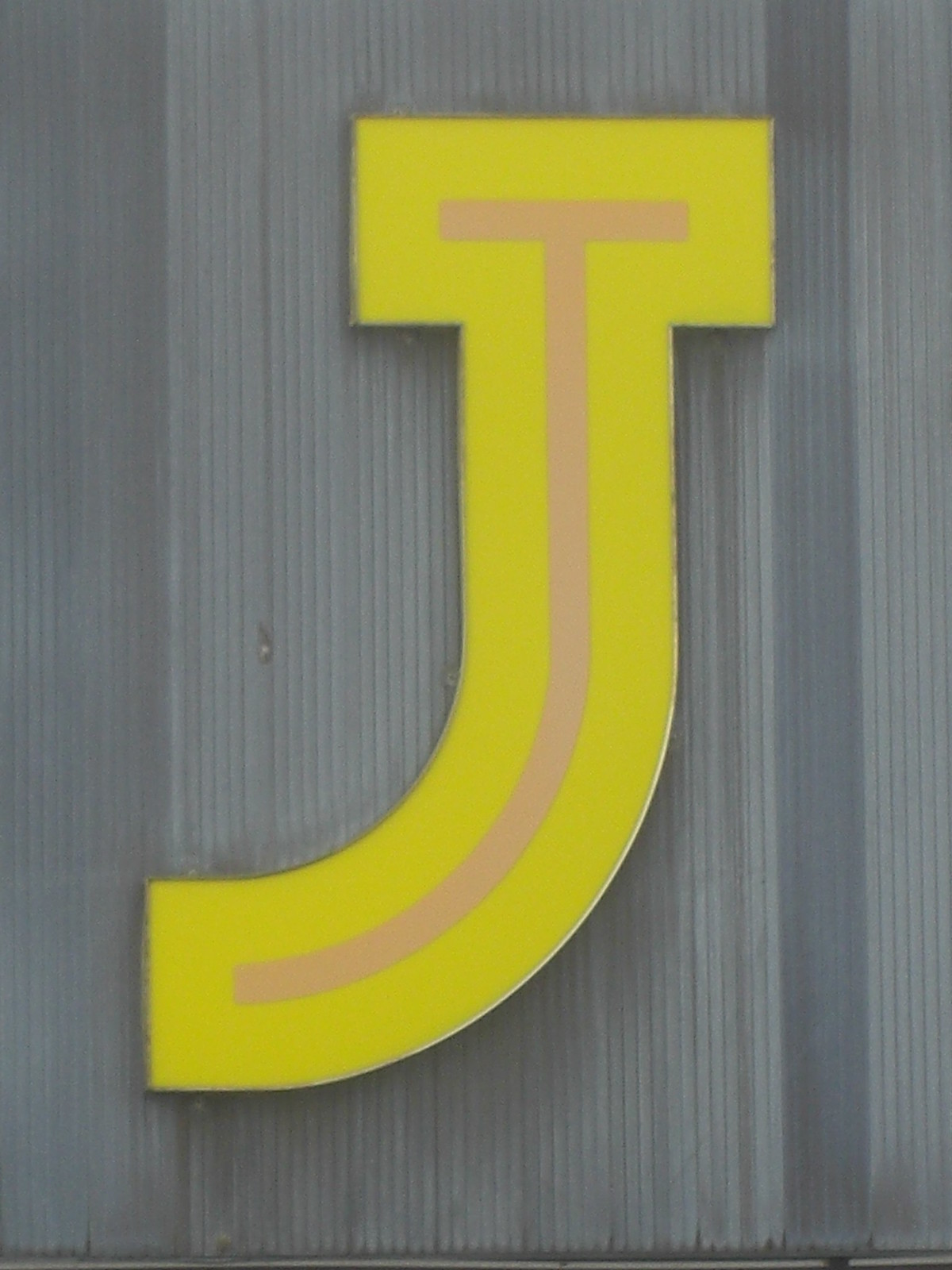This photograph depicts a large, capital J prominently displayed on the side of a gray corrugated metal building, possibly made of aluminum. The letter J, which appears to be made of plastic and potentially capable of lighting up, is painted a vibrant yellow. Within the hollow of the yellow J, there is a smaller J, also crafted in the same shape but colored a pinkish-peach hue. The photo is an extreme close-up, focusing solely on the letter J, which has a slight curve at the bottom, resembling a T that drifts leftward. At the base of the image, the metal wall shows a darker line, likely a water stain, providing a minor contrast to the otherwise uniform metallic surface.